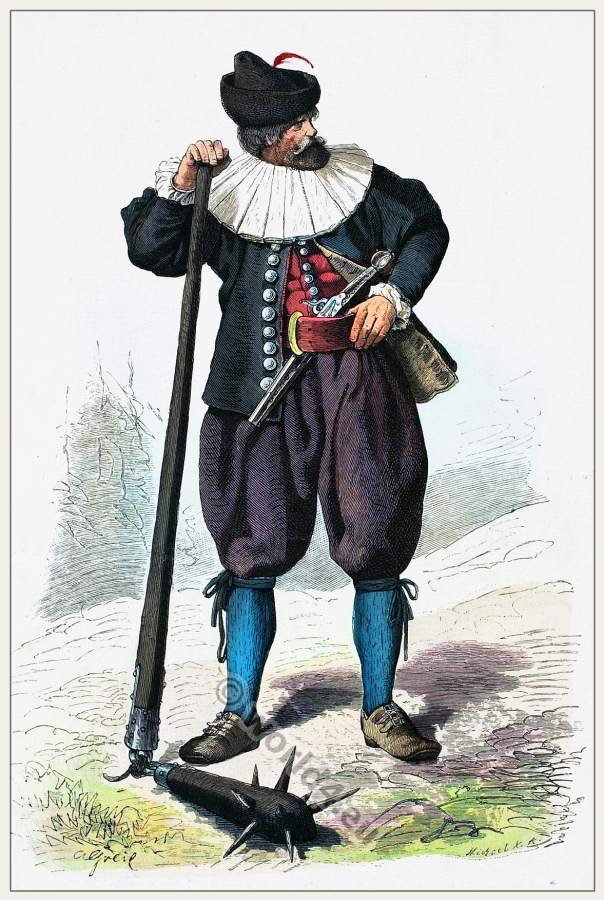The image is a colorful, vintage-style illustration in portrait orientation, likely resembling a color illustration from an old magazine or comic book. It portrays a man standing in an outdoor setting, dressed in period costume from possibly the 1600s Europe. He has a black beret hat adorned with a curled red feather, long black hair, a black beard, and a mustache. He wears a wide, white ruffled collar over a black jacket that is open at the front, revealing a red vest with silver buttons. A brick-colored belt with a gold buckle is around his waist, securing an old muzzle-loading pistol.

He is posed with his left hand resting on his belt below the pistol and his right arm raised, holding a large wooden weapon that’s almost as tall as he is. This weapon features a smaller spiked club attached by a short chain, resembling a deadly nunchuck with iron spikes. His pantaloons are dark gray and tied below the knees, complemented by blue knee socks and brown buckle shoes.

The background depicts a cream-colored hillside with light green patches in the foreground and indications of more hills behind him. There is a watermark across the bottom center of the image reading “US dot world for dot EU” in reverse, further indicating its vintage artwork style. This fierce, well-armed character, possibly a guard, appears ready for action.